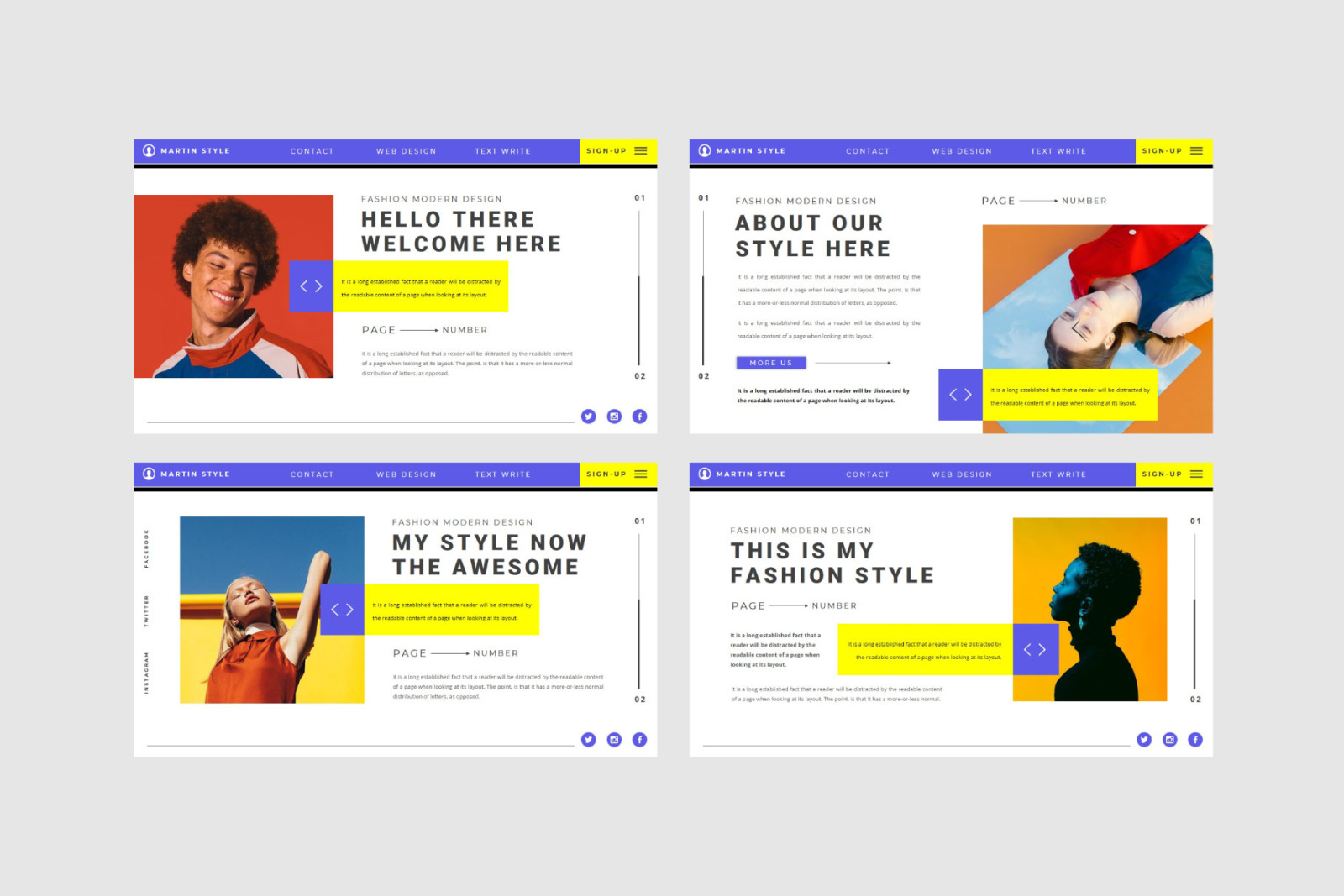The image features a gray background with a large central gray rectangle. Inside this large rectangle are four equally sized smaller rectangles, aligned in a 2x2 grid. Each of these smaller rectangles displays consistent design elements: a purple banner at the top with white text, and a white background beneath.

Upon closer inspection, the top left rectangle contains several textual elements, though some details are hard to decipher. The purple banner reads "Martin Style Contact Web Design." Below this, a black text section contains "Touch right, sign up." Further down, another header states "Fashion Model Design," followed by the text "Hello there, welcome here." The words "page number" are also present. The lower part is blurred, but the phrases "Long and Established" are somewhat readable.

The bottom left rectangle mirrors the layout of the top left, also featuring "Fashion Model Design" in its purple banner. Beneath, it says "My Style, Now, The Awesome." The phrase "It is Long, Established, Fat, Fat, A" is evident, though the rest is hard to read. The word "page number" appears again in this section.

The top right rectangle features the same purple banner with "Fashion Model Design" and identical layout. It contains the text "This is about our style here," and "page number." A purple box below states "More Us," and a paragraph mentions, "It is a Long, Established, Fat, that a reader will be distracted by the maybe readable context of the page when looking at its layout."

Lastly, the bottom right rectangle maintains the consistent design theme. The purple banner reads "Fashion Model Design" and below, it states "This is My Fashion Lifestyle page" followed by the text "advertisement number."

Overall, the image has a notable repetition and focus on the theme of fashion design, with slight variations in the content of each smaller rectangle. The text, although at times blurred, appears to be drawn from placeholder text commonly used in web design mockups.